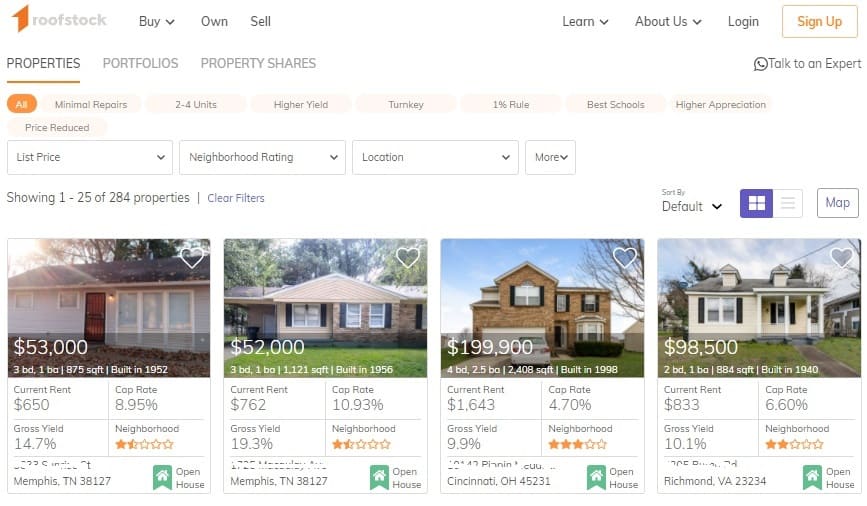The image is a screenshot of the Roofstock website, a platform dedicated to real estate listings. At the top of the screen, the "Roofstock" logo is displayed in gray, set against a white background. The logo features an orange design resembling both a roof and the number one. The main navigation menu includes options to Buy, Own, Sell, Learn, About Us, and Log In, with drop-down arrows for the Buy, Learn, and About Us sections. 

A prominent white "Sign Up" button outlined and labeled in yellow is visible. Below the main menu, there are further navigational tabs for Properties, Portfolios, and Property Shares, with Properties being highlighted. 

Filtering options are displayed below, including categories like All (highlighted in orange), Minimal Repairs, Two to Four Units, Higher Yield, Turnkey, 1% Rule, Best Schools, Higher Appreciation, and Price Reduced, all in pale orange. Additional drop-down menus are available for List Price, Neighborhood Ratings, Locations, and more. The screen shows that 1 to 25 out of 284 properties are being displayed, with options to clear filters and sort by Default via a drop-down menu. Users can also choose between Grid view (highlighted in purple with a four-pane window icon) and List view, with the current selection on Grid view. A Map option is also available.

Four property listings are shown:
1. The first house is priced at $53,000.
2. The second house is priced at $52,000.
3. The third house is priced at $199,900.
4. The fourth house is priced at $98,500.